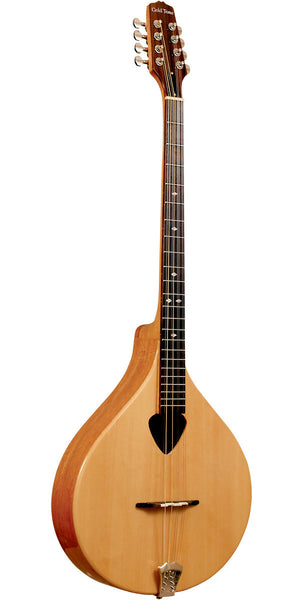This color photo features a meticulously crafted string instrument that appears to be a modern variation of a lute, closely resembling both a mandolin and an acoustic guitar. Unlike the classic hourglass shape of a typical acoustic guitar, this instrument boasts a distinctive teardrop-shaped body. The body is constructed entirely from wood, transitioning from a light brown hue on the front to darker brown on the sides. 

The instrument has eight strings, which are intriguingly in gold and silver, suggesting either artistic or functional nuances. The head of the instrument is dark brown and adorned with silver tuning knobs on the sides. At the top, there's a small golden inscription, although the text is unreadable due to its size. The neck is black with metallic silver frets and a black fretboard strip that contrasts beautifully with the woody tones of the body.

In the center of the light brown wooden body, there's a distinct, upside-down triangular black sound hole positioned just below the neck. Below this hole, a brown and white strip extends, guiding the strings to a small silver (or possibly gold) piece at the very bottom that secures the strings in place. The instrument is set against an all-white background, emphasizing its unique and detailed craftsmanship.